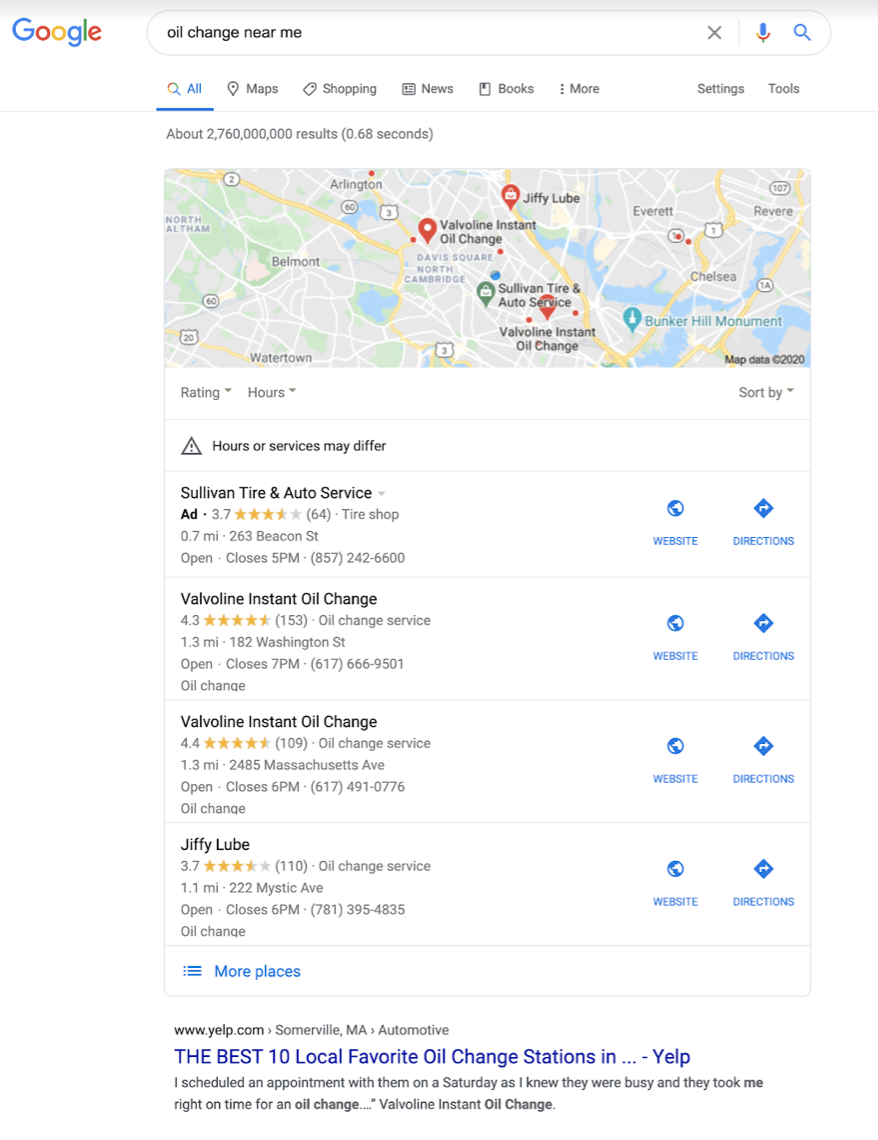The image depicts a search results page from a website called Kukli. The Kukli logo, characterized by its multicolored letters in blue, red, yellow, green, and red, is located at the top left corner of the page. The search query in the text box reads "oil change near me," accompanied by a microphone icon indicating voice search capability, and a search button.

Located below the search bar are navigation tags labeled as "All," "Maps," "Shopping," "News," "Books," "More," "Settings," and "Tools," with the "All" category currently selected and highlighted in blue. The search results indicate about 27,600,000,000 results found in 0.8 seconds.

A map is prominently featured on the page, displaying various locations for oil changes. Beneath the map, there is a "Places" section, offering the options to view "Websites" or get "Directions," both indicated by blue buttons.

The top search result is for "Sulevian Tyre and Auto Service," followed by "Valvoline Instant Oil Change" listed twice, and "Jiffy Lube." Further down, a "More places" button is also highlighted in blue.

At the bottom of the page, there is a link to Yelp.com, which showcases "The Best 10 Local Favorite Oil Change Stations" on Yelp, written in blue text. Additional descriptive text found below the Yelp link states, "I scheduled an appointment with them on a Saturday as I knew they were busy, and they took me right on time for an oil change," written in black.